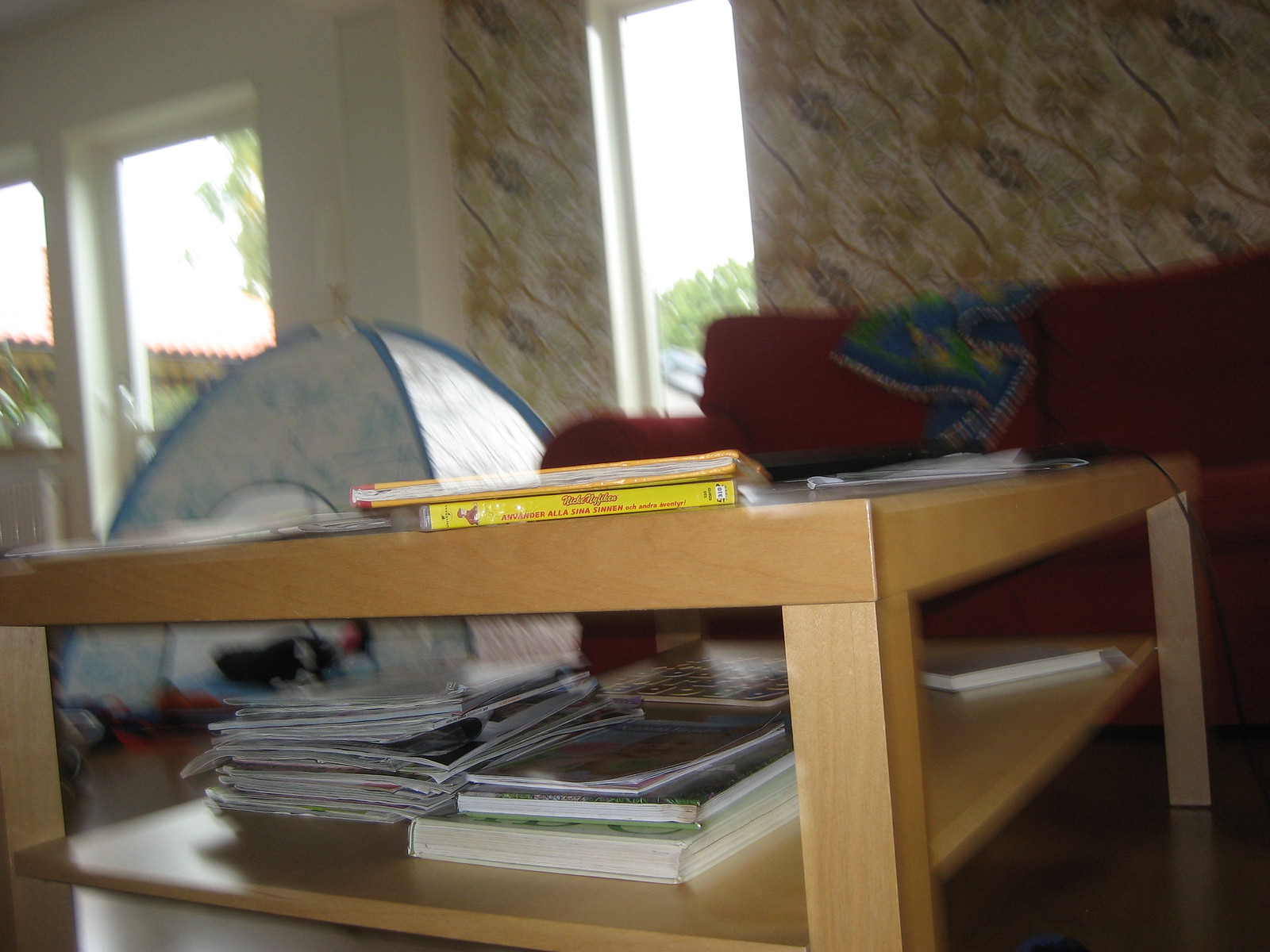The photograph showcases a cozy indoor setting centered around a wooden coffee table. The table's corner is prominently visible, adorned with an array of magazines and books spread across its middle section. At the top of the table, a couple of books are neatly stacked. In the background, a whimsical blue and white tent is set up, suggesting a playful space for a child within the home. To the right of the tent, a vibrant red sofa is draped with a blanket featuring bold blue, yellow, and green patterns. The backdrop reveals an eclectic mix of decor, with a brown and gold floral design embellishing the right-side walls, contrasted by white walls on the left. Additionally, two windows provide a glimpse of the exterior, adding a touch of natural light to the scene.